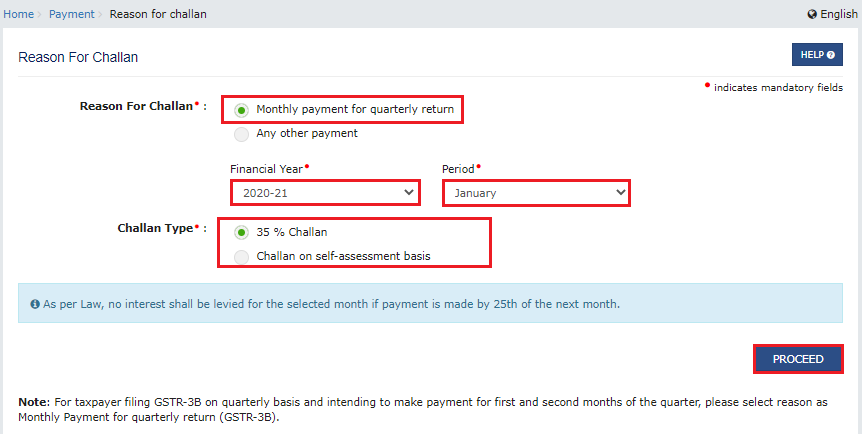The image is a screenshot of an online payment system interface. At the top, there is a gray title bar featuring several options on the upper left-hand corner, including a "Home" button, a "Payment" button, and a "Reason for Challan" button, with "Challan" spelled as "C-H-A-L-L-A-N." On the far right of the title bar, there is an "English" language option, accompanied by a global icon.

Below the title bar, a prominent white rectangular box displays the heading "Reason for Challan," with "Challan" written in uppercase letters. To the right of this box, there is a "Help" button in blue. Directly underneath, the text "Reason for Challan" appears again with an asterisk, indicating that it is a required field. 

Within this section, users can select the type of payment. Options include "Monthly Payment for a Quarterly Return" and "Any Other Payment." In this particular instance, "Monthly Payment for a Quarterly Return" is selected, highlighted by a red box and marked with a green dot.

Further down, there are fields for "Financial Year" and "Period." In this example, the financial year is set to 2020-2021, and the period selected is January, both of which are outlined in red boxes.

Lastly, the "Challan Type" section offers two choices: "35% Challan" and "Challan on Self-Assessment Basis." To the right-hand corner of the interface, a "Proceed" button is available for users to continue with their transaction.